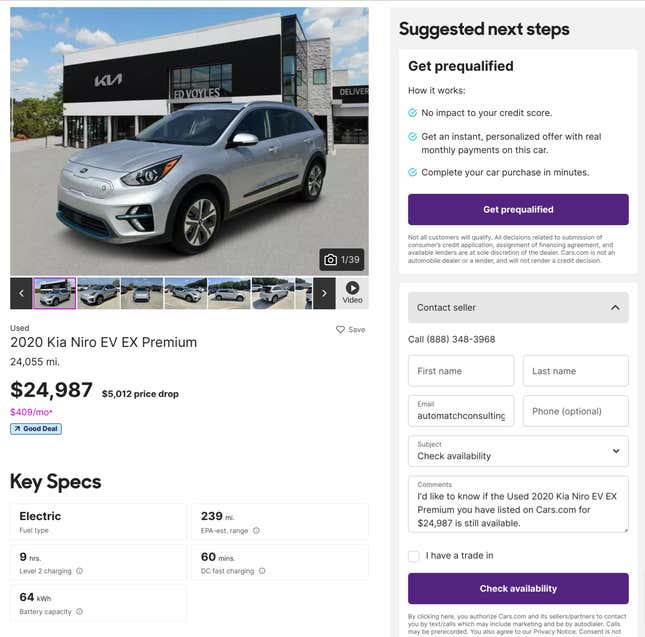This screenshot captures a detailed view of a Cars.com advertisement for a vehicle. Dominating the left portion of the screenshot is a large square thumbnail displaying an angled front view of the driver's side of the car. In the bottom right corner of this photo, a black box with a camera icon indicates "1 of 39." Below, a row of smaller square thumbnails showcases the vehicle from various perspectives, flanked by navigational arrows on both ends, and a square labeled "video" on the far right for scrolling purposes.

Directly beneath the images, the vehicle's details are displayed. The word "used" appears in small grey letters above the prominent listing of the vehicle model: "2020 Kia Niro EV EX Premium" rendered in bold black font. The mileage of 24,055 miles and the price of $24,987 are noted below, with an adjacent notice of a "$5,012 price drop." Under this, a purple text box shows the estimated monthly payment, and a blue box highlights it as a "good deal."

In the section titled "Key Specs," presented in bold black font, the advertisement lists various specifications of the vehicle within boxed formats. Adjacent to this, a large vertical box on the right is labeled "Suggested Next Steps," also in bold black text. This section includes options such as "Get Pre-Qualified," with a link to "How It Works" and a prominent purple bar at the bottom stating, "Get Pre-Qualified."

Further down, a white box labeled "Contact Seller" offers a drop-down menu with the default option set to "Contact Seller," and contains the seller's phone number for direct calling. Below this, text boxes invite input for first name, last name, email, and phone number. A "Subject" field defaults to "Check Availability," followed by a comments box. At the very bottom, a small checkbox allows users to indicate if they have a trade-in. Concluding the section is a large purple button labeled "Check Availability," positioned at the bottom right of the page.